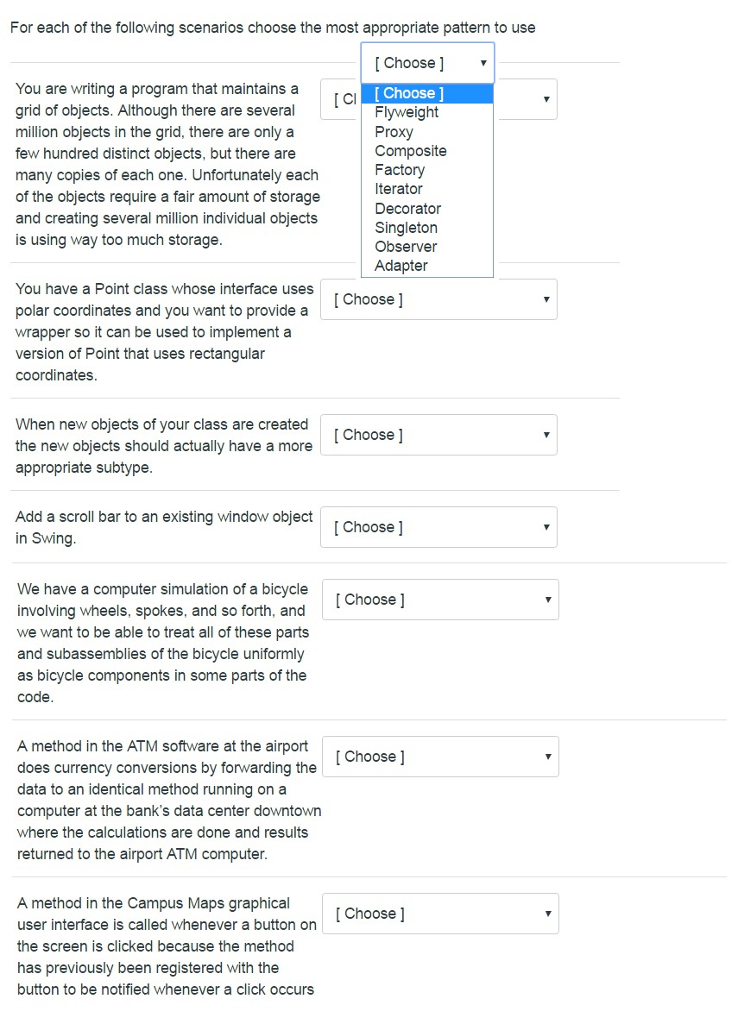Here is a detailed and cleaned-up caption for the image you described:

---

The image is a screenshot of a questionnaire interface, likely viewed on a phone or computer, intended for software developers. At the top, there is an instructional sentence that reads, "For each of the following scenarios, choose the most appropriate pattern to use." The main interface is divided into two columns: on the left, each question is presented within a paragraph, and on the right, a drop-down menu allows users to select their answers.

The questionnaire comprises seven questions of varying lengths. For example, the fourth question is relatively brief and states, "When new objects of your class are created, the new objects should actually have a more appropriate subtype." Another question asks, "Add a scroll bar to an existing window object in Swing." These inquiries suggest the focus is on object-oriented programming, design patterns, and user interface elements.

The overall theme of the questionnaire appears to be evaluating the appropriate application of design patterns in various programming scenarios, making it a specialized tool for web developers or software engineers to assess their skills in handling development tasks.